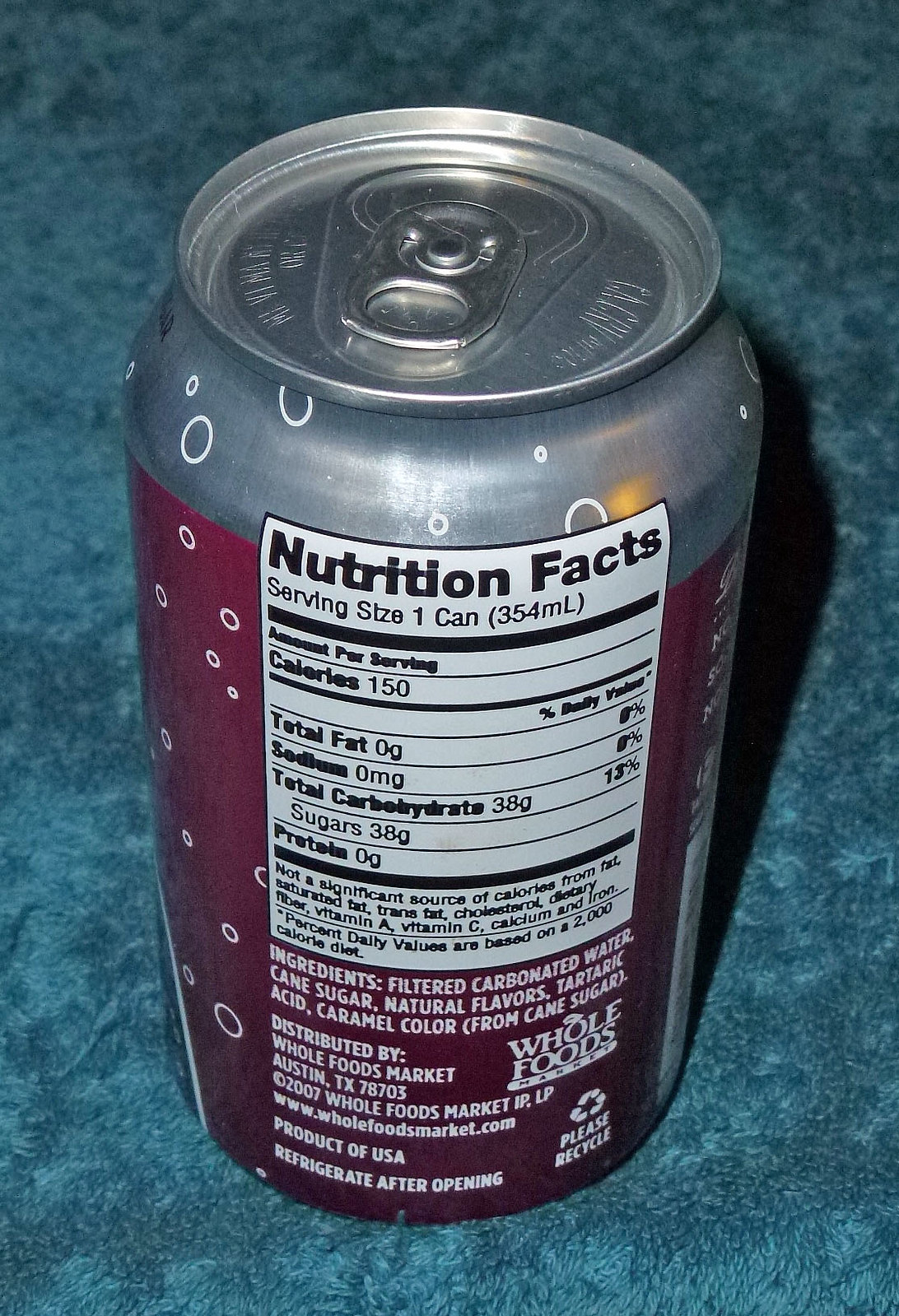**Caption:**

An aluminum soda can sits on a green countertop. The can features a maroon label adorned with small white circles, and an aluminum pop-top lid designed to be pulled up, pushing a small ring down to open. The front of the can displays the nutrition facts, including a serving size of 1 can (354 milliliters) and 150 calories. It indicates 0 grams of total fat (0% DV), 0 milligrams of sodium (0% DV), 38 grams of carbohydrates (13% DV), and 38 grams of sugar. The label notes that the drink is not a significant source of calories from fat, saturated fat, trans fat, cholesterol, dietary fiber, vitamin A, or vitamin C. The ingredients list includes filtered carbonated water, cane sugar, natural flavors, and caramel color derived from cane sugar. The soda is distributed by Whole Foods Market, based in Austin, Texas, 75705. The label also encourages recycling and notes that the product is made in the USA. It advises to refrigerate after opening.